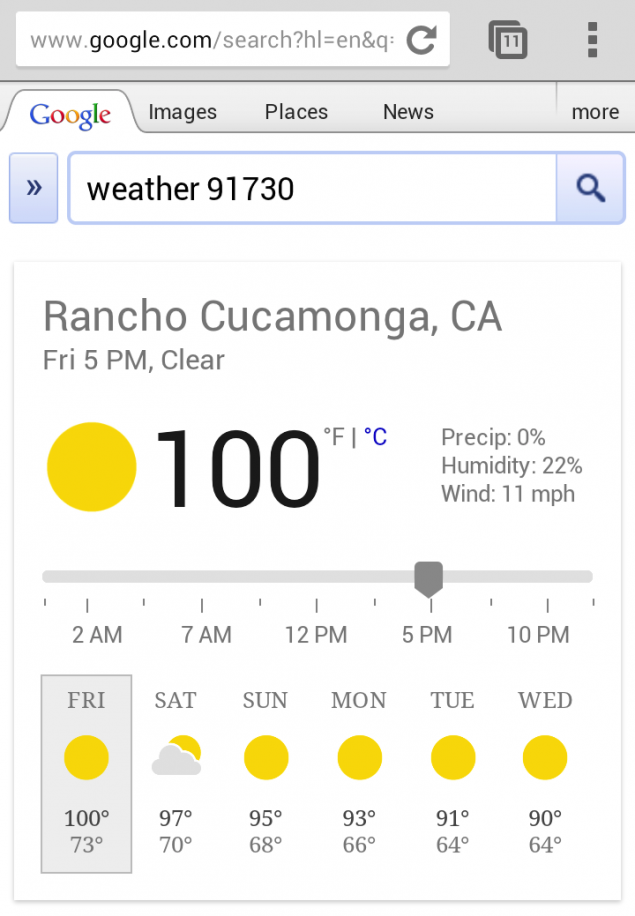The image captures a Google search result for the weather in Rancho Cucamonga, California (zip code 91730). It displays detailed weather information for Friday at 5 PM, indicating clear skies and a sweltering temperature of 100 degrees Fahrenheit. The conditions reveal zero precipitation, 22% humidity, and wind speeds of 11 mph. 

Just below this, a timeline bar provides a breakdown of the weather at different times throughout the day, specifically at 2 AM, 7 AM, 12 PM, 5 PM, and 10 PM. Additionally, a forecast for the upcoming days is displayed:
- **Friday**: Sunny, with a high of 100 degrees and a low of 73 degrees.
- **Saturday**: Partly cloudy, with a high of 97 degrees and a low of 70 degrees.
- **Sunday**: Sunny, with a high of 95 degrees and a low of 68 degrees.
- **Monday**: Sunny, with a high of 93 degrees and a low of 66 degrees.
- **Tuesday**: Sunny, with a high of 91 degrees and a low of 64 degrees.
- **Wednesday**: Sunny, with a high of 90 degrees and a low of 64 degrees.